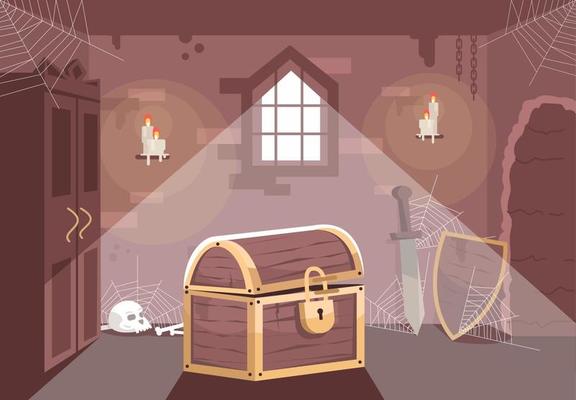The image is a cartoon drawing of a room, possibly an abandoned or haunted house. Dominating the center, an unlocked brown treasure chest with gold trim and a gold lock casts a shadow on the gray floor. A stream of light filters through a barred window in the back wall, creating a pyramid-like beam that illuminates the scene. The back wall is a blend of light brown and purple-brick, contrasting with the darker brown ceiling.

To the left stands a tall closed cabinet with gold handles, spiderwebs in its upper corners. On the ground beside it, a skull and a couple of bones lie covered with cobwebs. On the right side of the chest, a sword leans against the wall next to a shield, also draped in cobwebs. Additionally, lit candles mounted on the walls drip wax, enhancing the eerie ambiance. To the far right, an arched entryway signifies a partially dug-out wall or cavernous entry, adding to the mysterious and possibly sinister setting.